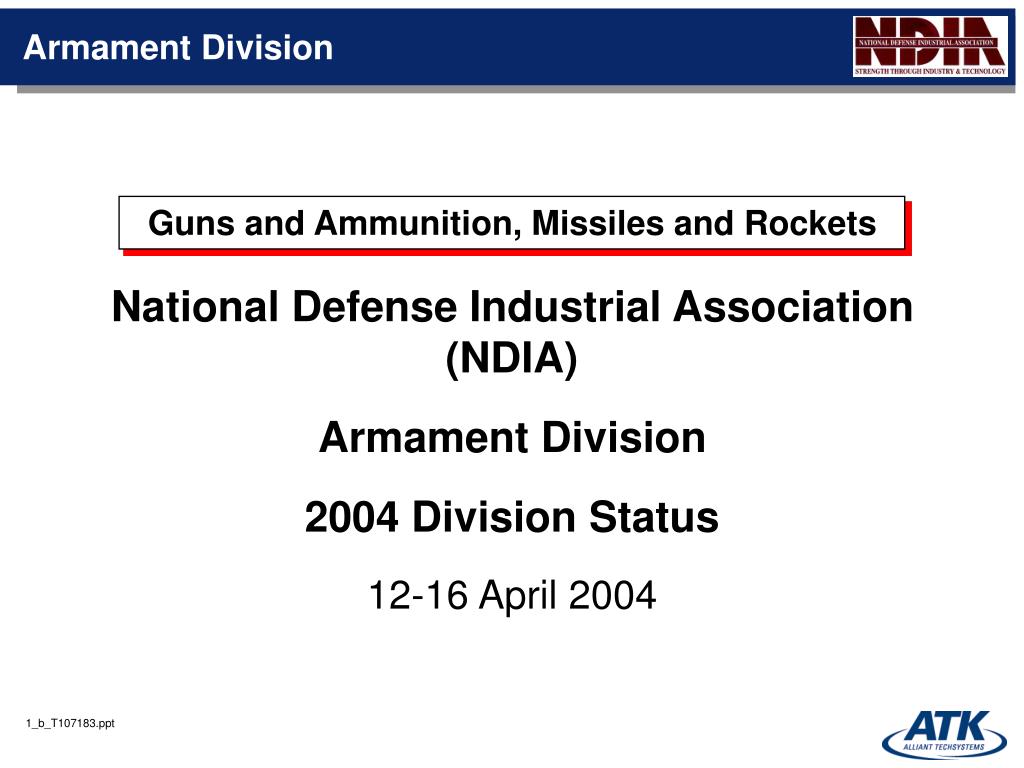The slide features a dark blue title bar at the top with white text on the left reading "Armament Division" and the NDIA logo in red on the right. Below, a text box with a red shadow on the right side contains black text stating "Guns and Ammunition, Missiles and Rockets." Beneath this, black text on a white background lists "National Defense Industrial Association (NDIA)," followed by "Armament Division," "2004 Division Status," and "12-16, April 2004." In the lower right corner, there is an ATK logo with some illegible text below it, enclosed in a circle around the base of the letters.